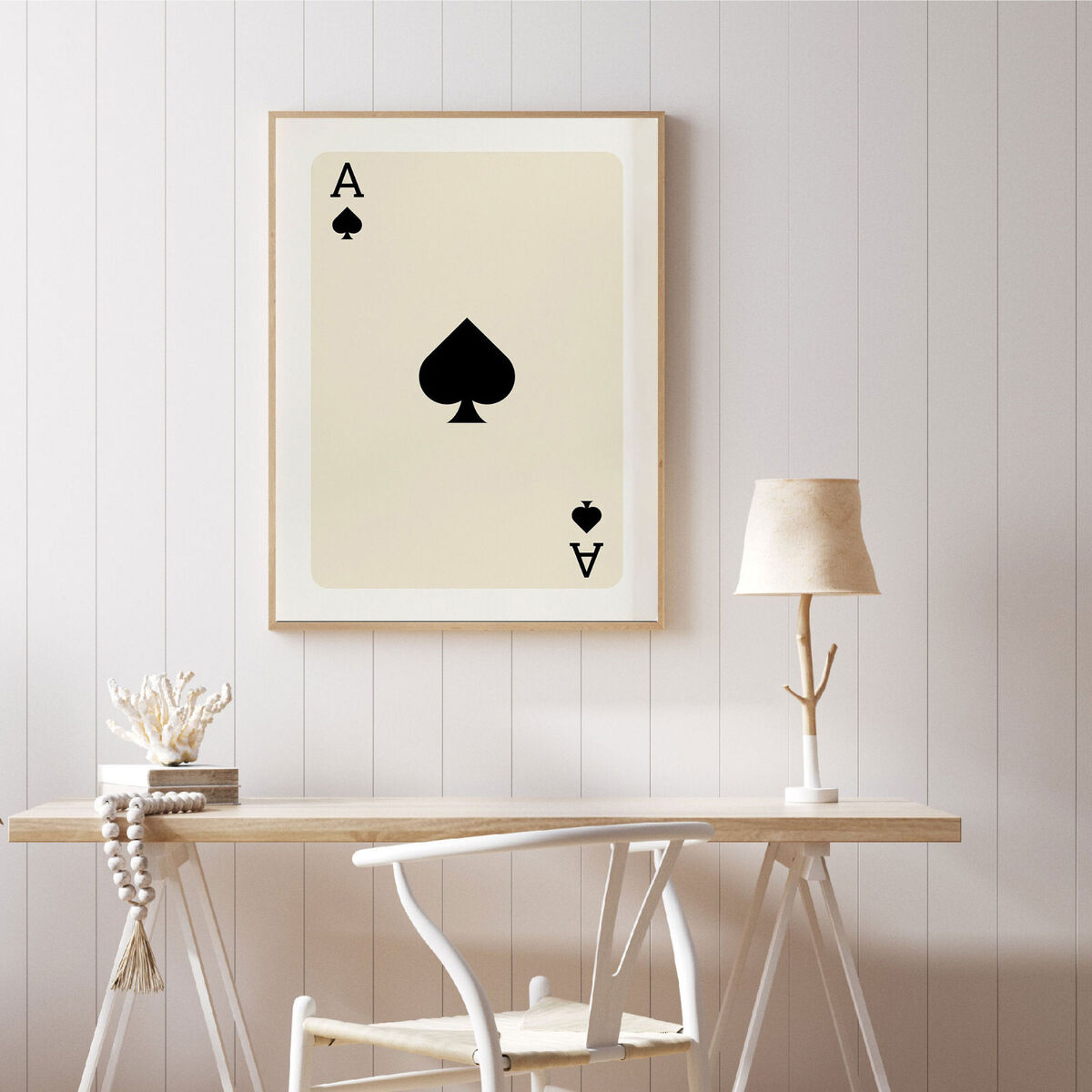In this photograph, likely taken inside a home or studio, the main focal point is a framed artwork featuring the Ace of Spades playing card. The artwork is displayed prominently on an off-white, vertically paneled wooden wall, and it is encased in a beige frame with a white border. Below the framed card is a small table with white legs arranged in an A-pattern, and a natural wood tabletop. Accompanying the table is a white woven chair. A distinctive lamp, crafted from a tree limb and topped with a slightly crumpled white lampshade, sits on the table. To the left, a decorative piece resembling a white leaf spread and a large beaded necklace with white pearls drapes over the table-edge, alongside an artistic fragment of ocean coral. The entire setting boasts cohesive shades of white and beige, creating a serene and cohesive aesthetic akin to a high-end furniture or home decor catalog.